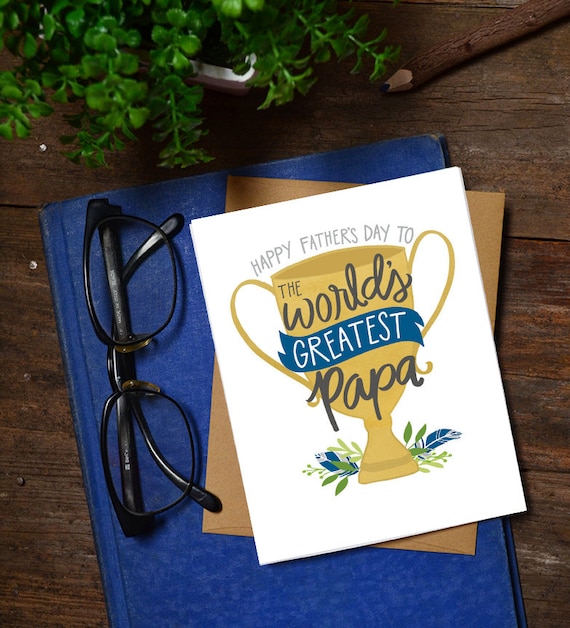This image showcases a charming arrangement on a brown wooden table. At the center is a white card with the title "Happy Father's Day to the World's Greatest Papa" prominently displayed. The card features a golden trophy cup with ring-shaped handles, with the word "Greatest" highlighted on a blue section of the cup. This card rests on a brown envelope which in turn is placed atop a blue hardcover book. To the left of the card, there is a pair of black frame glasses without lenses. Above this central arrangement, a green plant in a white container adds a touch of fresh greenery. This carefully curated scene on a wooden surface beautifully combines a heartfelt message with thoughtful details.